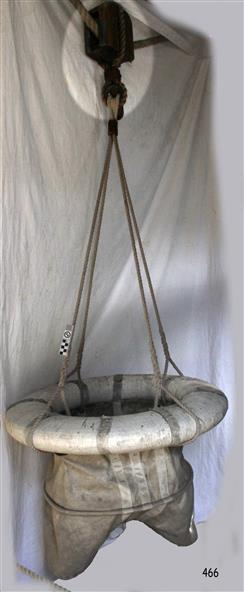This photograph depicts a hanging flotation device against a white curtain backdrop. The device, resembling a life preserver, is primarily white and gray with a yellow, sine-wave patterned bottom edge, where the left and right sides are longer, and the middle section dips. Suspended by a black or gray fastener, this preserver is attached to a coat hanger or similar apparatus via brown ropes configured in a triangular format. Each rope's end forms a loop that encircles the preserver. At the base, a circular brown fabric with tan vertical stripes extends inwards from the lifesaver. The prominent number "466" is conspicuously overlaid at the bottom right corner of the image, hinting at potential significance. The overall composition suggests a nautical theme with an emphasis on safety and functionality.